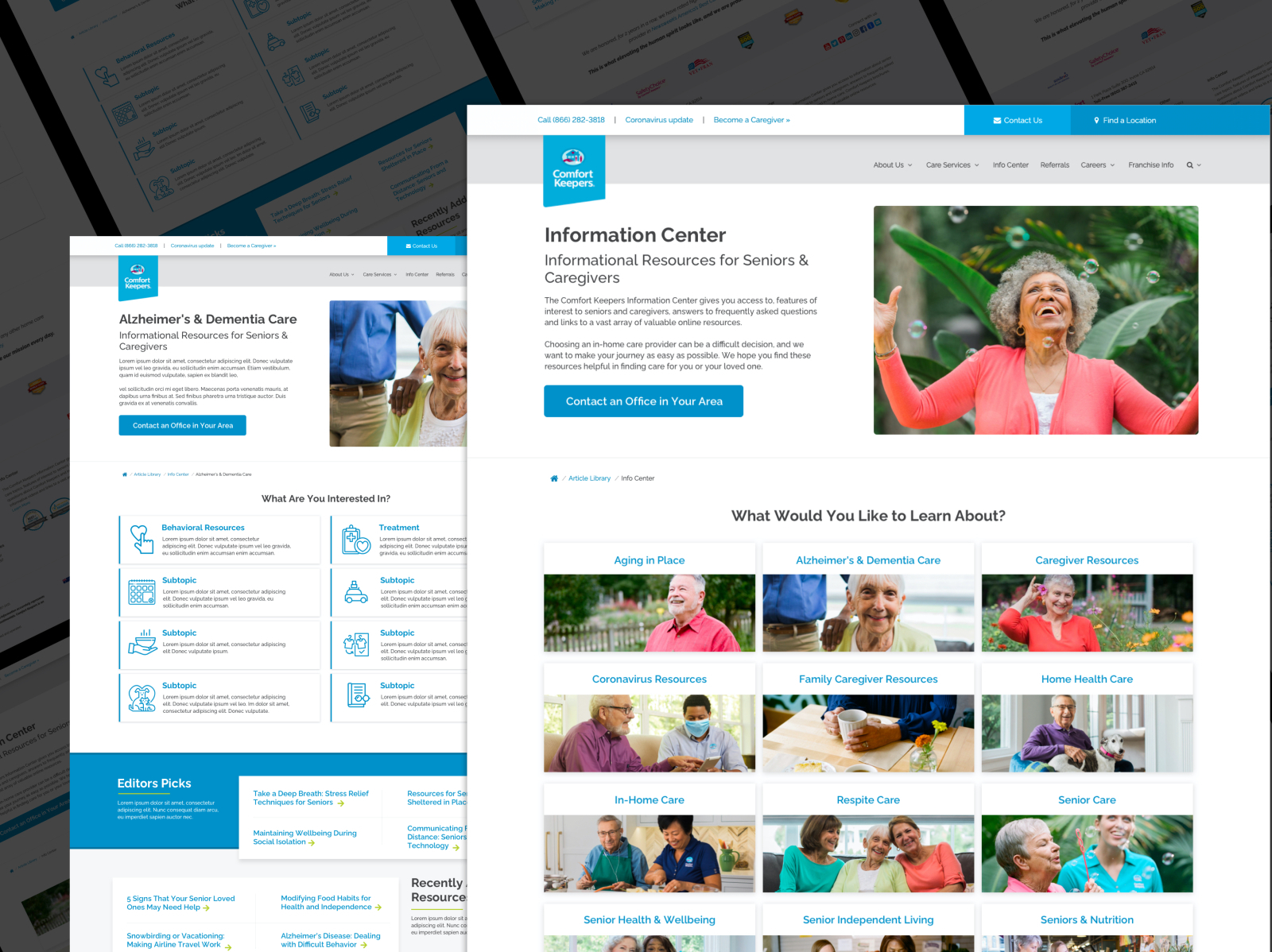The image features a black background with a white paper sheet in the foreground. Across the top of the sheet, blue print is visible, followed by a blue box. Below the blue box, there is a gray box containing black print and a small blue box in the corner. Prominently displayed in black text is the title "Alzheimer's and Dementia Care," accompanied by a picture of an elderly gray-haired woman standing beside a man. The sheet includes a short article and a blue box beneath it.

On the left side, there are four small boxes, each accompanied by blue lines. Similarly, on the right side, there are another set of four small boxes with blue lines next to them. A large blue box further down the sheet is labeled "Editor's Picks," featuring smaller blue captions within it. Following this, a gray box appears with the heading "Recently," detailing information about resources in blue print.

On the right side of the image, the design transitions from white at the top to shades of light and dark blue. A long gray strip runs vertically, housing various captions and additional small blue elements. The text "Information Center Informational Resources for Seniors and Caregivers" is marked in black print on a white section, with a blue button labeled "Contact an Office in your area" nearby. An image of another gray-haired woman looking up at bubbles is included.

Further down, the section prompts "What Would You Like to Learn About," listing topics such as Aging in Place, Alzheimer's and Dementia Care, Caregiver Resources, Family Caregiver Resources, Home Health Care or In-Home Care, Respite Care, Senior Health and Well-Being, Senior Independent Living, and Senior Nutrition.